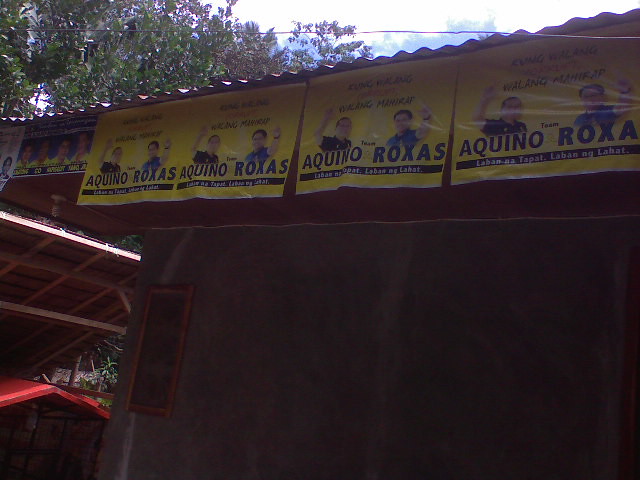This color snapshot, taken outdoors in low light, showcases the side of a concrete building with a shadowy bottom portion, leaving little detail visible there. Above, an awning made of wood extends out, with the image capturing part of its beams bathed in sunlight on the left-hand side. Under this awning, four yellow posters are hung side by side. Each poster features the head and shoulders of two smiling men, one in a blue shirt and the other in a black shirt, both appearing to have black hair and likely being white. They are depicted waving, and though the text is somewhat blurry and not in English, the legible parts read "Aquino Roksas." In the background, at the top of the image, the sky and outlines of trees are visible. The posters seem to be part of a promotion for a team or event related to "Aquino Roksas," though specifics remain unclear.